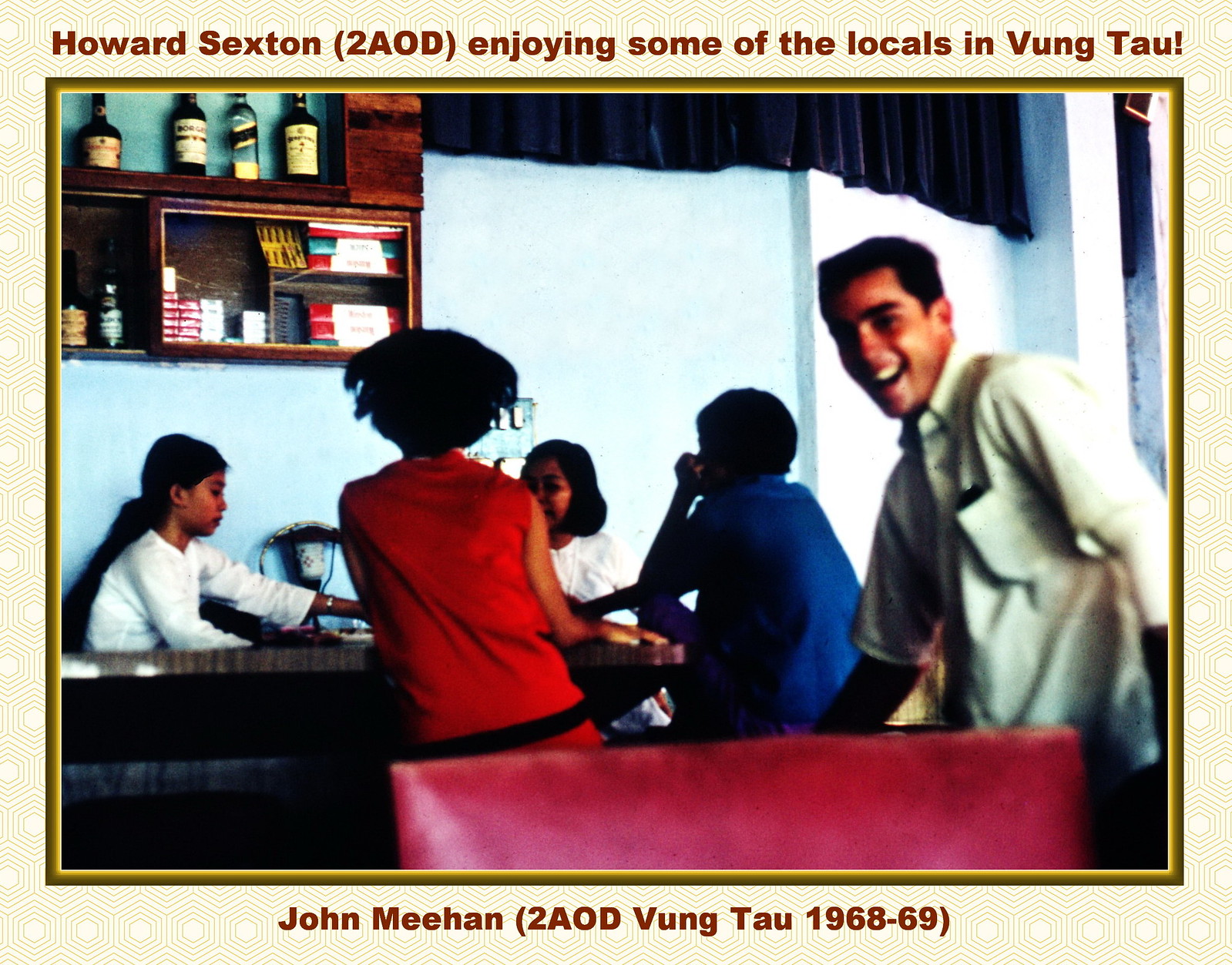In the image, Howard Sexton (2AOD) is seen enjoying the company of locals in Vung Tau, with the event dated 1968-69. The scene takes place in a bar, where Howard, easily recognizable by his green shirt with a pocket, is smiling at the camera. He sits on a stool next to a woman in a red dress, who in turn sits beside a lady in a blue dress, and another in white. The backdrop is light blue, and in the background, there is a glimpse of a red booth or chair back. The bar area is well-stocked, with a cabinet of liquors on the wall, and a lamp on the table. There are also blue curtains hanging near a window behind them. A bartender, a woman with her hair tied in a ponytail and wearing a white shirt, is seen behind the counter, occupied with serving drinks. Additionally, there are cigarettes stored in a case on the wall. The image is framed, with vibrant details and a scene bustling with convivial interaction.